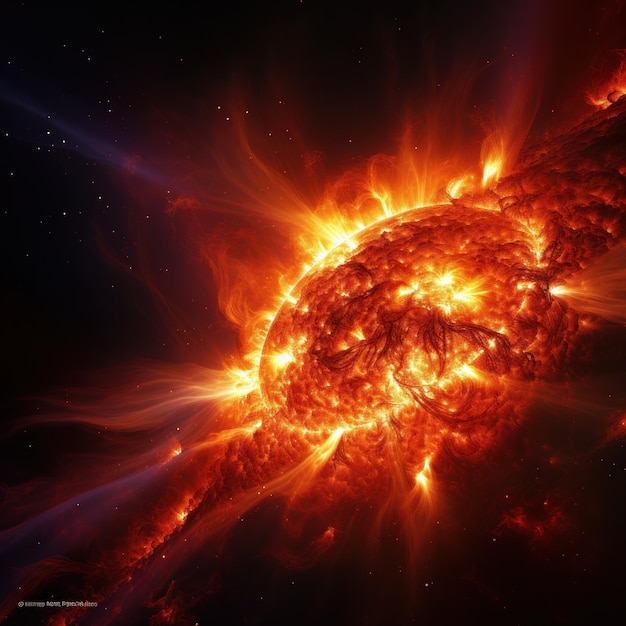The image depicts a dramatic scene in space with a black night sky scattered with tiny white stars as the background. Dominating the center of the image is a massive, bright, and fiery explosion, likely a representation of the sun or a similar celestial event. The explosion features an oval shape with an intense orange-red hue, surrounded by fiery tendrils and billowing molten smoke extending outward in all directions. The incandescent explosion extends diagonally towards the bottom right, with a more cloudy shape concentrated below and around the right of the central mass. Along the top, the vibrant, elongated tendrils of fire appear to reach outwards, creating a dynamic and chaotic effect. Additionally, there is a yellow outline encircling most of the explosion, adding depth and intensity to the scene. In the bottom left corner of the image, some indistinct white writing is visible.